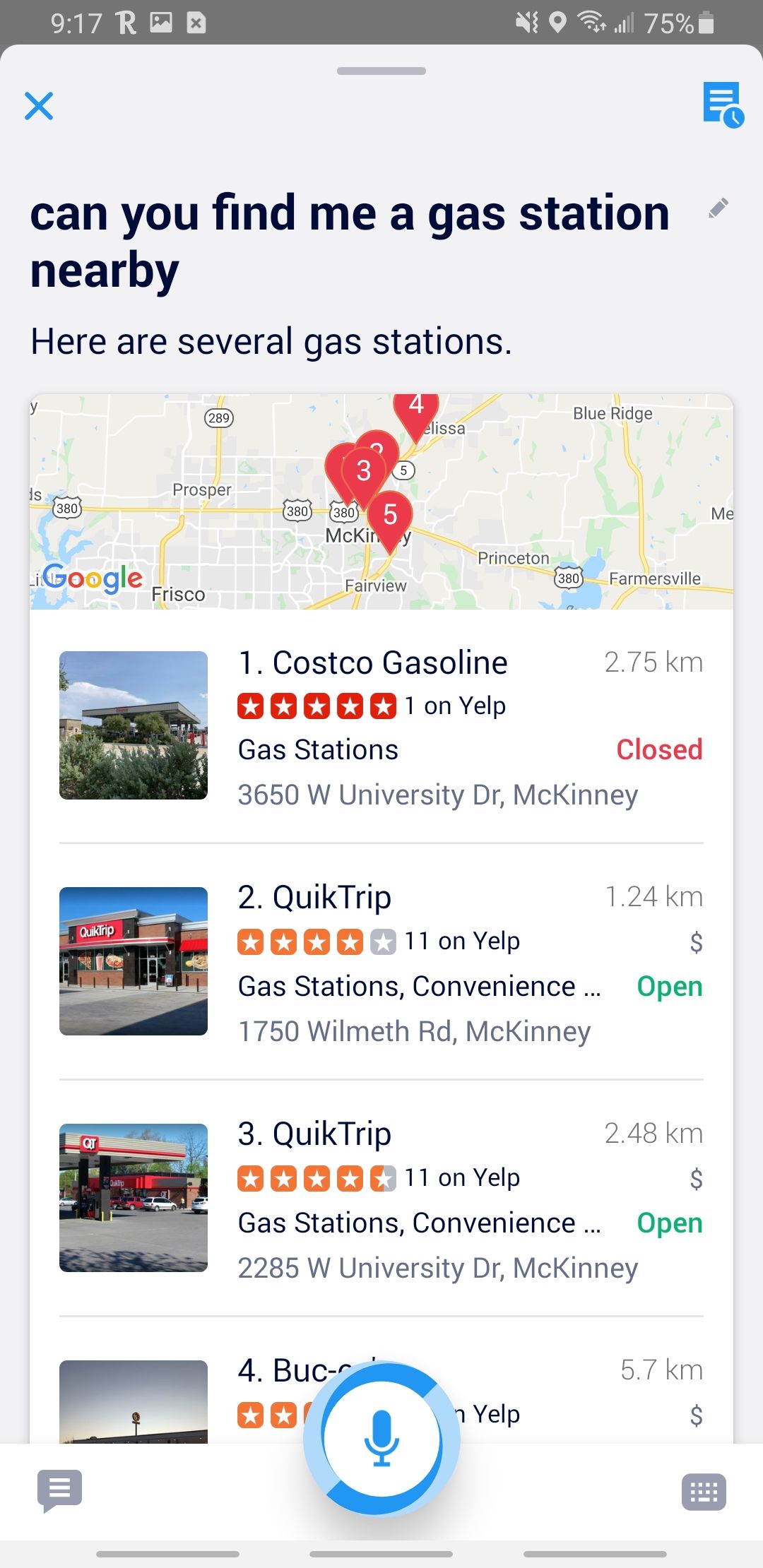A smartphone screen displays a voice-activated search query for nearby gas stations. At the top, in black text, it says "Can you find me a gas station nearby?" The resulting search information is overlaid on a map displaying several towns including Fairview, Prosper, Frisco, Princeton, Blue Ridge, and Farmersville. There are five numbered red checkpoints marking the gas stations on the map.

1. Coastco Gasoline, located 2.75 km away at 3650 W University Dr, McKinney, is rated the number one gas station on Yelp. It has a 5-star rating but is currently closed.
2. Quick Trip, ranked 11 on Yelp and situated on Wilmeth Road, is open and has a 4-star rating.
3. Another Quick Trip, located on W University Dr, has a 4.5-star rating.
4. The details of the last gas station are partially obscured by a blue and white record button at the bottom of the screen.

Additionally, there are interface elements displayed: a message button on the bottom left and a keyboard button on the bottom right.